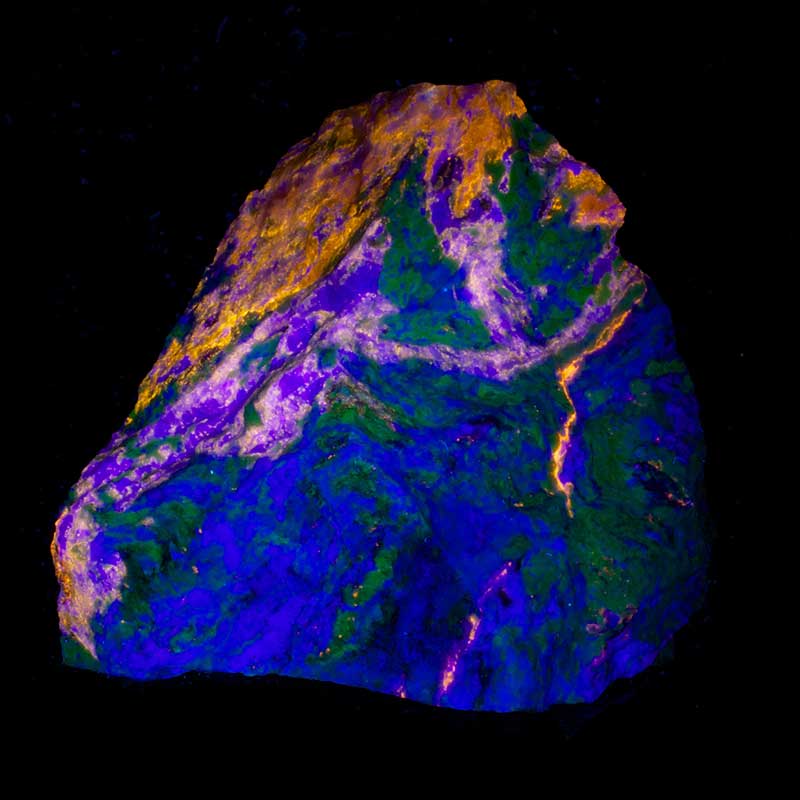The image captures an abstract art piece or possibly a photograph of a mineral that has been digitally enhanced with vibrant lighting. The centerpiece resembles a jagged rock face with a textured, multi-layered composition. The rock's base is dominated by intense electric blues and dark greens, creating a vivid, almost glowing effect. Midway through the rock, streaks of purples and violets emerge and intertwine, creating a dynamic transition. The upper portion of the rock transforms into an orangey-amber hue, with prominent gold tones that blend into light blue stains. The overall effect is reminiscent of a lava flow, cascading from the orangey, gold-dominated top down through the vibrant purples and blues, and settling into the striking electric blue base. The rock is set against a black or transparent background, accentuating its vivid, almost otherworldly appearance.